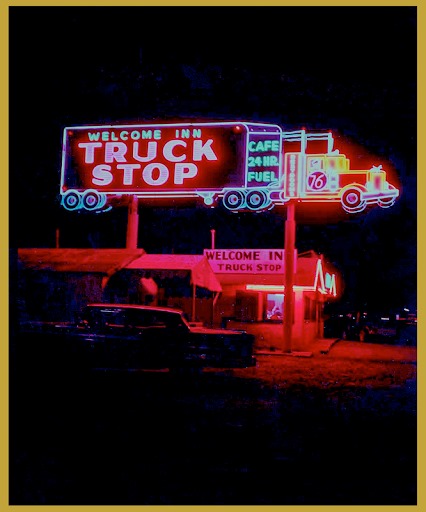The photograph captures a nostalgic truck stop from the 1950s or 1960s, cloaked in nighttime darkness, with the only light provided by vivid neon details. Dominating the scene is a strikingly large sign shaped like an 18-wheeler truck, almost spanning the length of the building. This sign is an explosion of color with neon lights in blue, green, red, pink, purple, and yellow. The truck's trailer displays "Welcome Inn Truck Stop" in bold red and green neon, while "Cafe 24-Hour Fuel" is prominently lit up in blue. On the truck's cab, the number "76" is displayed in bright red, reminiscent of Union 76 gas stations. The truck's tires and outlines are traced in blue neon, creating an arresting visual against the pitch-black night. Parked in front of the truck stop is the silhouette of an older car from the 1960s, adding to the retro ambiance. The building itself appears as a one-story structure with a few windows, subtly illuminated by the red hue of the neon lights.